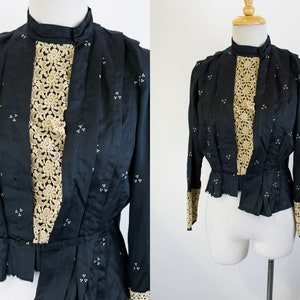The image displays two photographs of a white mannequin showcasing an antique jacket, set against a plain white background. The photo on the left is a close-up, highlighting the intricate details of the black jacket, which features a small triangle print and a pleated bonus leading into a band around the waist. The jacket has a small stand-up collar and a rough hem, suggesting it may have once been attached to a skirt. Beneath the jacket, or as part of its lining, is a beige lace with open work that peeks through, creating a mesh-like texture. The right-side photograph offers a wider view, revealing the mannequin's full upper body dressed in the same jacket. This perspective shows the jacket's long sleeves, which are trimmed with the same beige lace found underneath. The mannequin itself is headless and limbless, emphasizing the garment displayed. The ensemble appears to be prepared for fitting, reflective of a historical tailor shop setting.